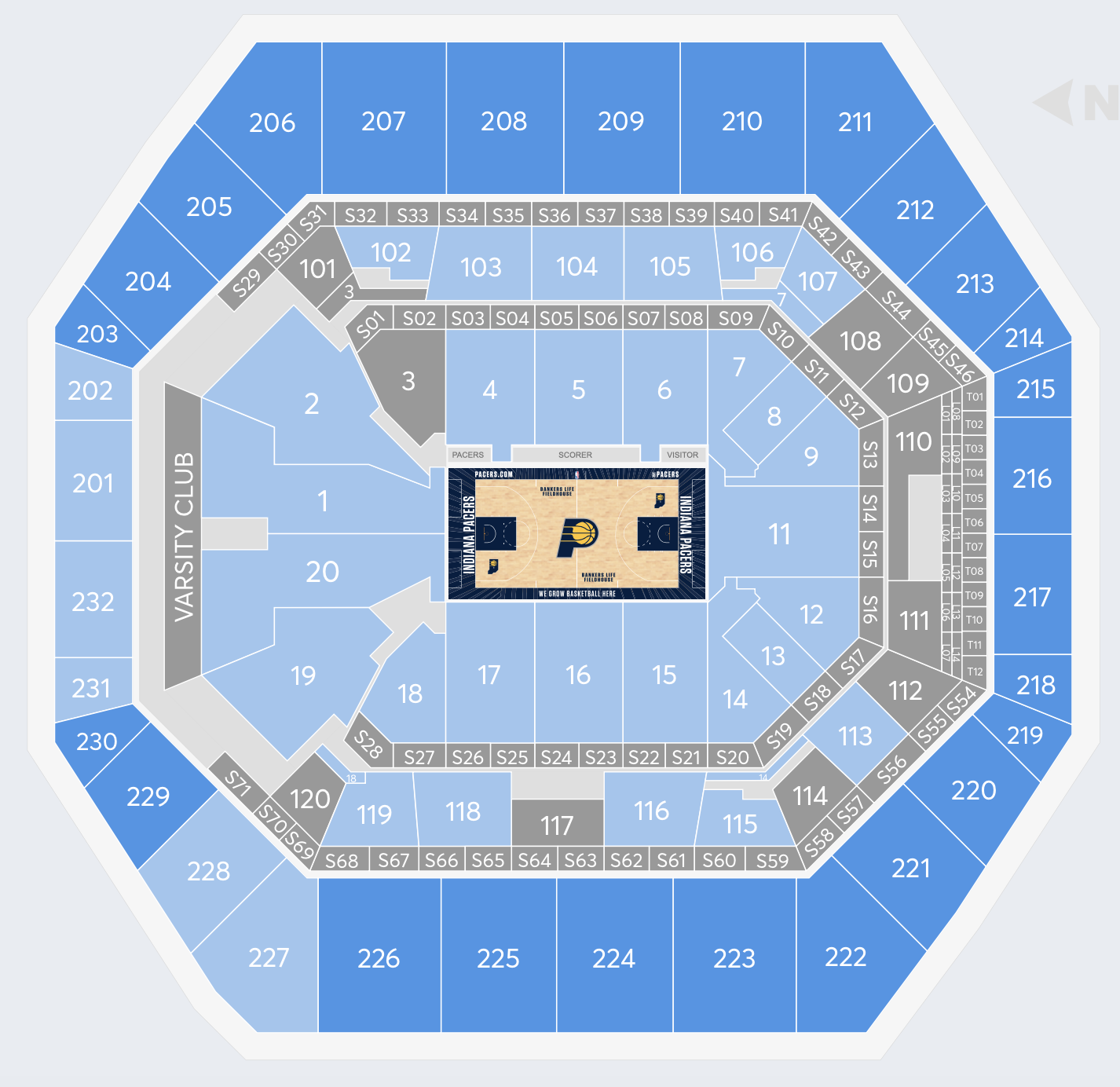The image showcases the seating arrangement for a basketball game featuring the Indiana Pacers. The layout details various designated areas, including sections for the Pacers, the scorers, and the visiting team. Prominently displayed in white lettering behind each hoop is "Indiana Pacers." The basketball court itself is brown, adorned with the team’s logo—a stylized "P" with a basketball forming the "O."

Surrounding the court is an octagonal seating arrangement, with sections in light blue, gray, and darker blue. Each seat is marked with white numbers. The background outside the octagonal arrangement is a light dove gray color. A notable feature is the "Varsity Club" inscription on one of the gray sections at the upper edge of the image.

The detailed high-resolution image also appears to be used for an online platform, likely to assist fans in selecting their seats by providing a clear view of the seating chart and its details.